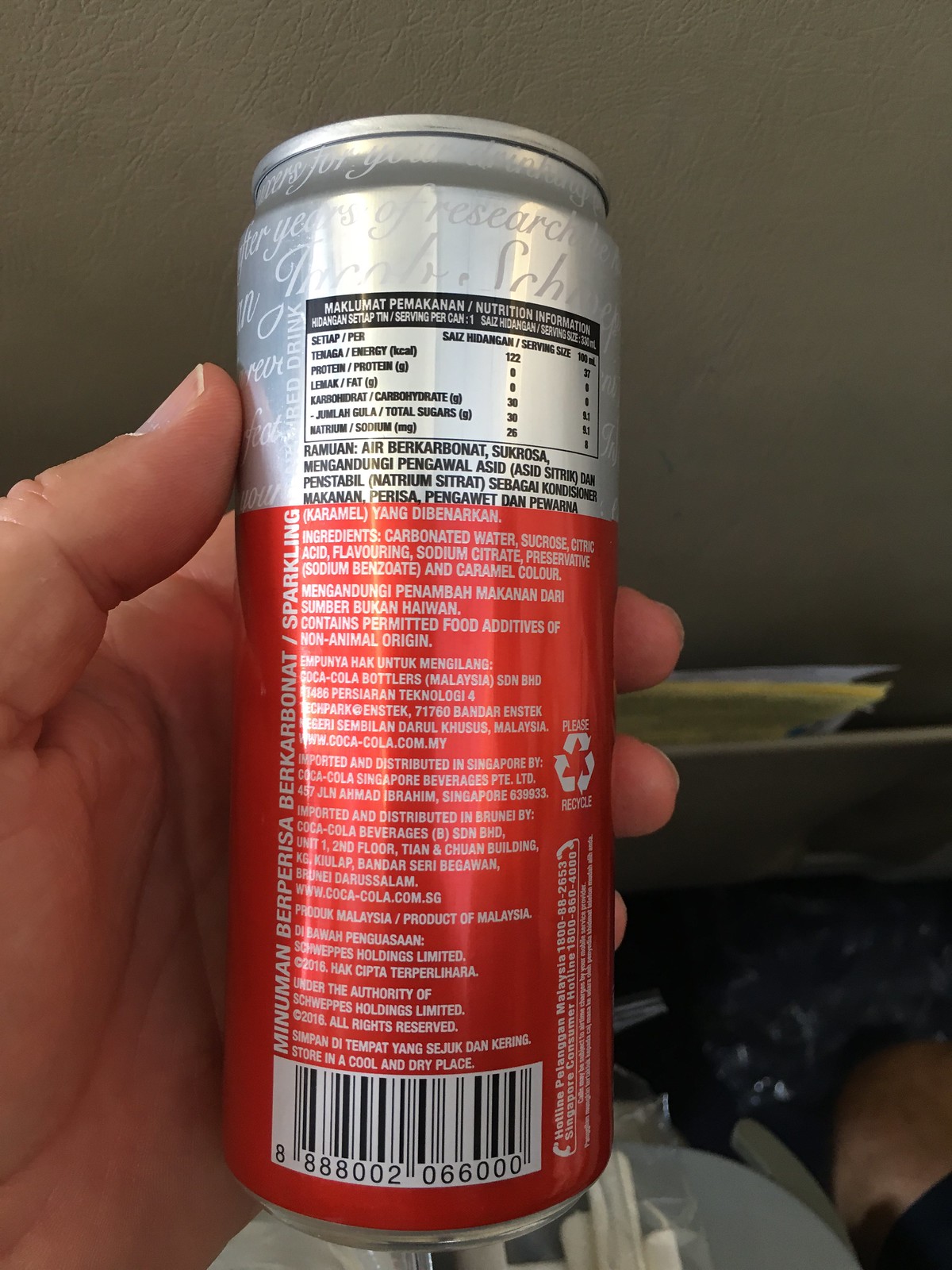A close-up photograph showcases a can held in the left hand of an individual, with the thumb and part of the fingers visible. The can, predominantly red for its lower two-thirds and silver at the top, displays a mix of both foreign and English text. The back of the can features a prominent barcode at the bottom. Above it, there are ingredients listed: carbonated water, sucrose, citric acid, flavoring, sodium citrate, preservative, sodium benzoate, and caramel colors. Some text is written in white and red, including a line stating "Contains permitted food additives with non-animal origin." A recycling symbol and the instruction to 'store in a cool and dry place' are also present. Intriguingly, the words "MINUMAN BERPERISA BERKARBONAT / sparkling" run vertically along the red portion, hinting at the beverage's foreign origin, possibly Indonesian. Nutrition facts occupy the silver section, where one can discern partial words and phrases, such as "years of research" and names starting with "Jacob" and "SCH," though they are partly obscured. The can urges to "please recycle," further underlining its global appeal and environmental considerations.